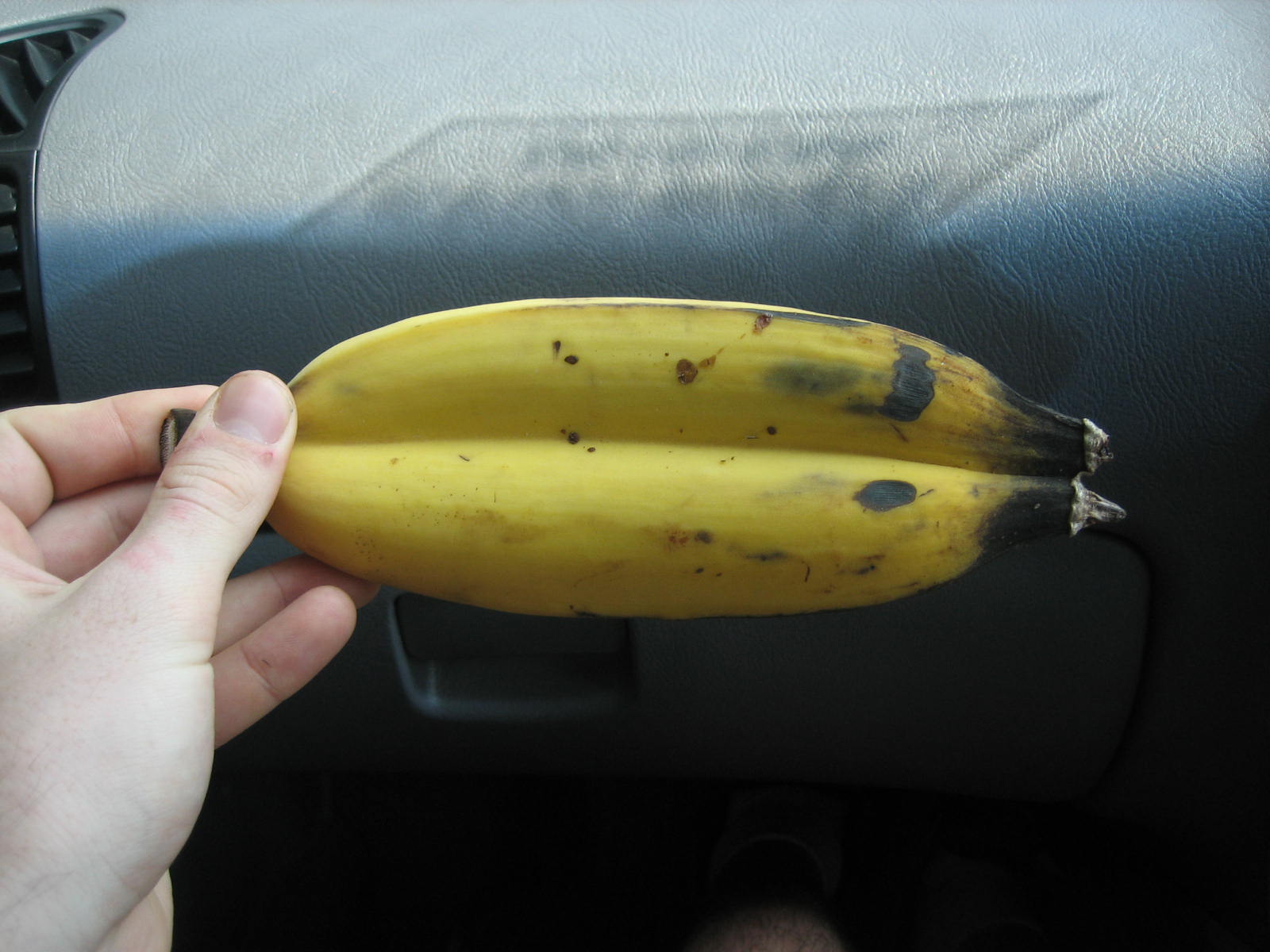In this rectangular photograph, a human hand holds two bananas that have merged together, giving the illusion of a single elongated banana. The bananas, held by their stem, are oriented horizontally with the stem pointing to the left and the base to the right. The left hand of the person grips the stem with their thumb, index, and middle fingers. The banana peels exhibit a yellow hue scattered with black spots, with more pronounced black discolorations at the stem and base.

The setting appears to be the interior of a car, specifically the passenger side. Visible in the background are elements of the car's dashboard, colored gray and made to mimic leather, complete with various textured surfaces. On the lower part of the dash, there is the glove compartment latch, alongside a triangular-shaped air vent positioned in the top left corner. Additionally, a sticker reflected on the dash hints at its location on the windshield. The overall scene captures a unique and detailed moment within the vehicle’s interior.